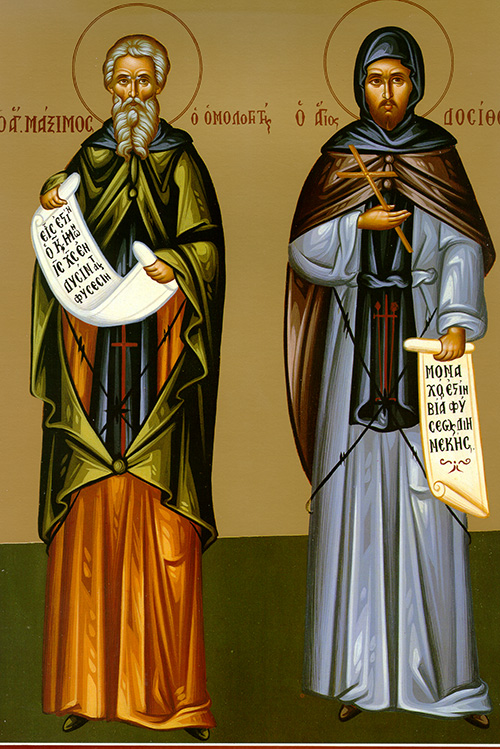The image is a beautifully detailed painting of two religious figures, likely drawn from the Orthodox tradition and linked to St. Mary Byzantine Catholic Church. The background is predominantly gold, shifting to black at the bottom to suggest the floor. Both figures are haloed, denoting their sanctity.

On the left stands Venerable Father Maximus the Confessor, identifiable by his long gray-white beard and hair. He is dressed in a gold robe that transitions to orange towards the lower half, and holds a white scroll with black lettering. A green shawl drapes down to his knees, revealing a red cross at the front.

To his right is another holy man, distinguished by a blue hood over his head, a brown shawl, and a long silver robe. He, too, holds a scroll inscribed with black writing and carries a cross. Both figures exude an aura of reverence and spiritual authority, captured poignantly in this Orthodox icon's detailed and colorful artwork.